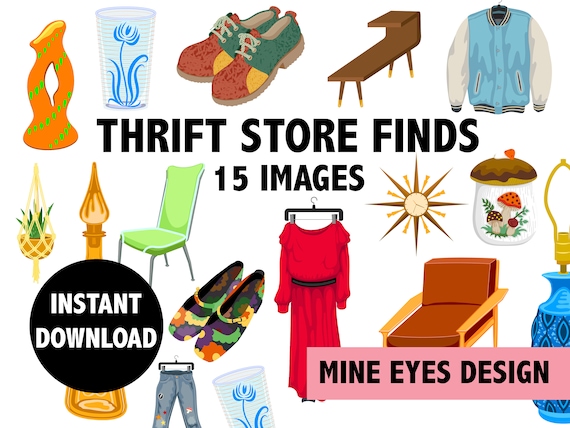The image displays a digitally illustrated collage titled "Thrift Store Finds" centered in bold black text against a white background, stating there are 15 images. Surrounding the title are various colorful renderings of typical thrift store items. These include a red dress on a hanger, a varsity jacket, a mid-century leather armchair, women's and men's shoes, a pair of jeans, a candle holder, a vase with purple dots, a glass with a painted blue flower, a lamp, a cookie jar filled with mushrooms, a potted plant, and a table. Each illustration is presented in a clip-art style, offering a vibrant array of colors and detailing distinct characteristics. A black circle near the bottom left corner says "Instant Download" in white text, suggesting the images are available for easy download. In the bottom right corner, a pink rectangle with black text reads "Mine Eyes Design," indicating the creator or source of these downloadable assets. The collection is likely intended for use in advertisements, social media, or digital content, capturing the eclectic essence of a thrift store.